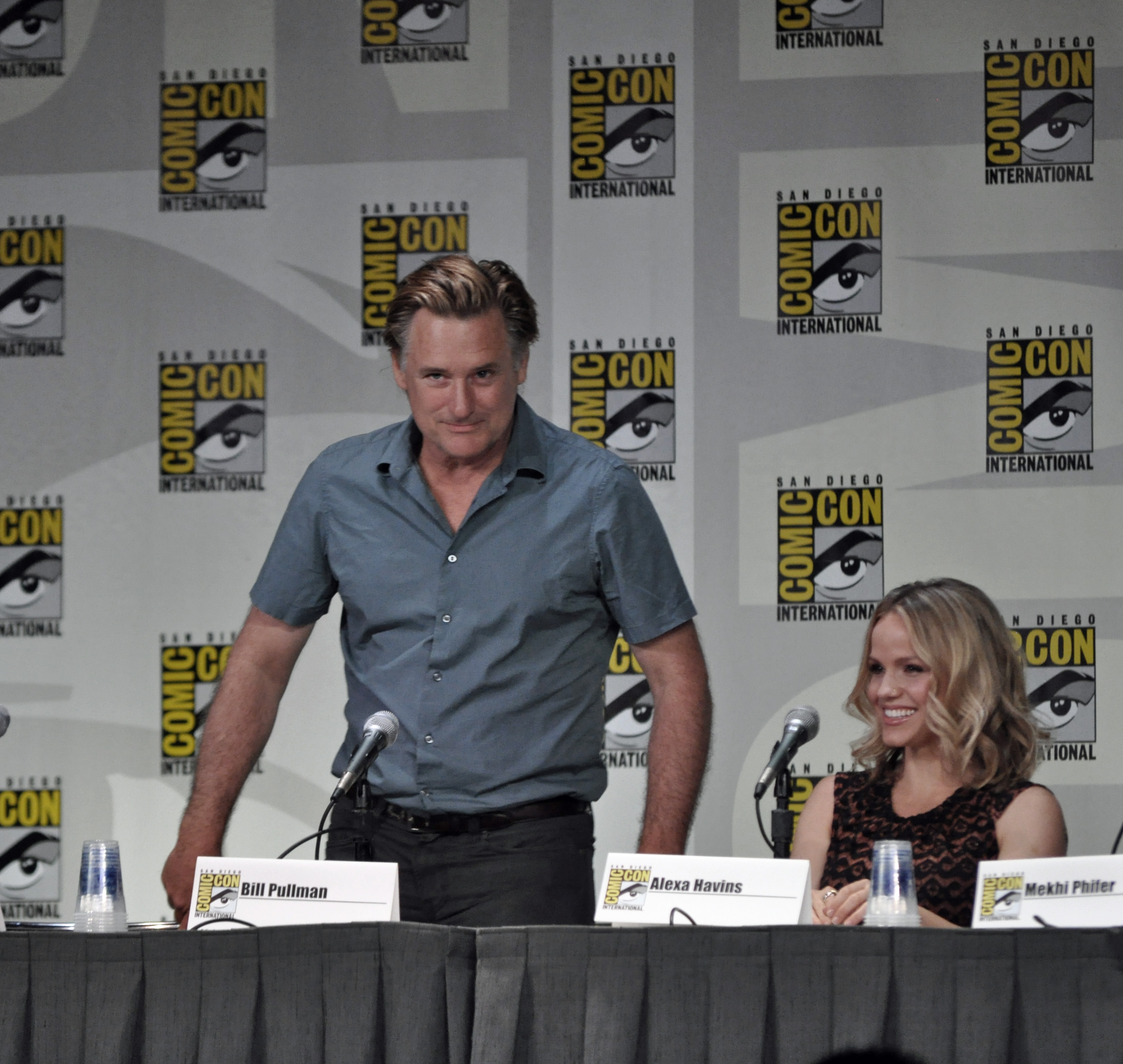In this detailed photograph taken at San Diego Comic-Con International, two prominent individuals are seated behind a table covered with a gray curtain-like tablecloth. In the foreground on the left side of the table, there is a stack of upside-down plastic cups. Three white name cards made up of folded pieces of paper are positioned on the table, labeled with black text: Bill Pullman, Alexa Havitz, and Mekhi Pfeiffer. 

The individual on the left is a standing man, identifiable from the waist upward. He sports dark-colored pants secured with a brown leather belt and a short-sleeve dark gray shirt with clear acrylic buttons. With slicked-back hair and his gaze directed towards the middle of the photo, his posture suggests engagement in the ongoing panel discussion. 

Adjacent to him on the right is a seated woman with dyed blonde hair, smiling broadly to reveal her teeth. She is dressed in a sleeveless dress that features a brown and black pattern. Her name card reads Alexa Havins, though the text from some accounts appears as Alexa Havitz. 

Microphones are set up on the table, indicating that they are likely participating in a panel, answering questions about a TV show or similar content. The background reveals a banner that confirms the event location as San Diego Comic-Con International, reinforcing the convention ambiance. The image's colors are dominated by shades of gray, dark gray, white, and yellow, further highlighting the professional and formal atmosphere of this significant gathering.